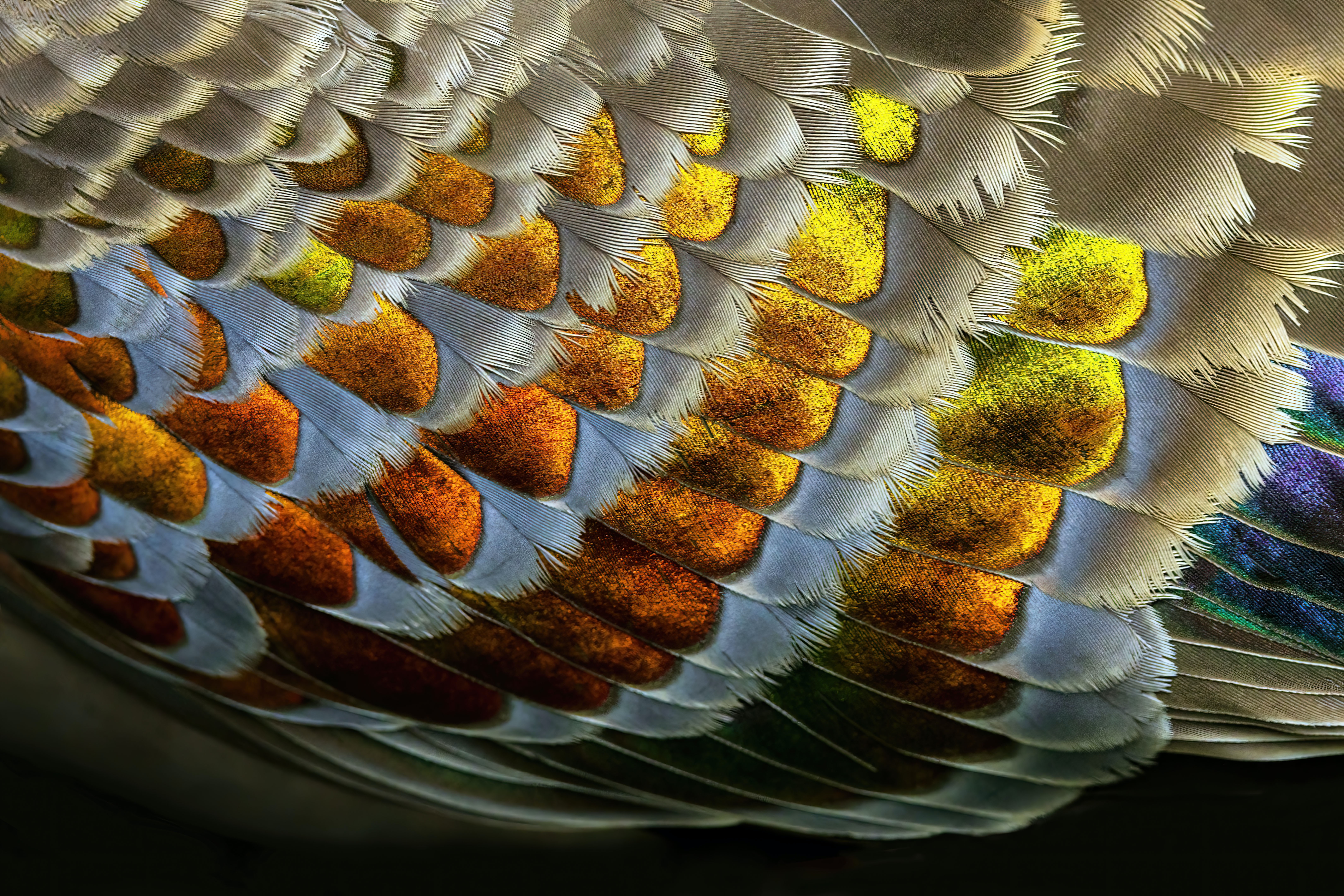This image appears to be a highly detailed, close-up photograph or an AI-generated depiction of bird feathers, resembling an art piece you might find in a museum. The feathers are intricately laid out in a partial section, set against a dark, black background that makes them appear to glow. Each feather has a base color that transitions from off-white and beige at the bottom to silver towards the top. The quills of the feathers remain white, contrasting with vibrant hues within the feathery plumes. The feathers exhibit a rich array of neon, metallic colors including deep purples, iridescent blues, radiant greens, bright oranges, and yellows. These colors form a rainbow-like arrangement across the feathers, contributing to a soft, yet luminous iridescence. This intricate pattern suggests a peacock feather-like appearance, with the light seemingly emanating from underneath, enhancing the glowing effect.